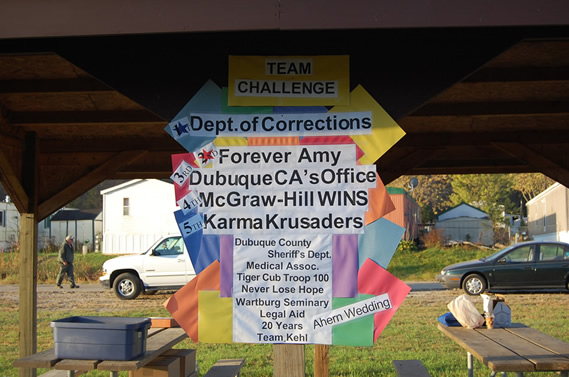The image depicts an outdoor picnic area featuring a dark brown wooden gazebo roof supported by wooden posts. Below the gazebo, there are two brown wooden picnic tables. The table on the left has a blue bin on top, while the table on the right is laden with several blue and white bags and a white box.

Prominently displayed in the middle is a sign detailing various affiliations and messages. It starts with "Team Challenge" on a white background, followed by "Department of Corrections" in black text. Additional text on the sign includes phrases like "Forever Army," "Dubuque CA's Office," "McGraw-Hill Winds," "Karma Crusaders," "Dubuque County Sheriff's Department," "Medical Association," "Tiger Group 100," "Never Lose Hope," "20 Years," and "Team Keeley." The papers surrounding the sign are of various colors, including yellow, blue, red, purple, orange, and a lighter blue.

In the background, a man in a gray or green outfit can be seen walking. There is a white truck and a green car parked nearby, along with some white houses and a yellow trailer with a green roof. The scenery includes green trees and grass, adding to the outdoor atmosphere.